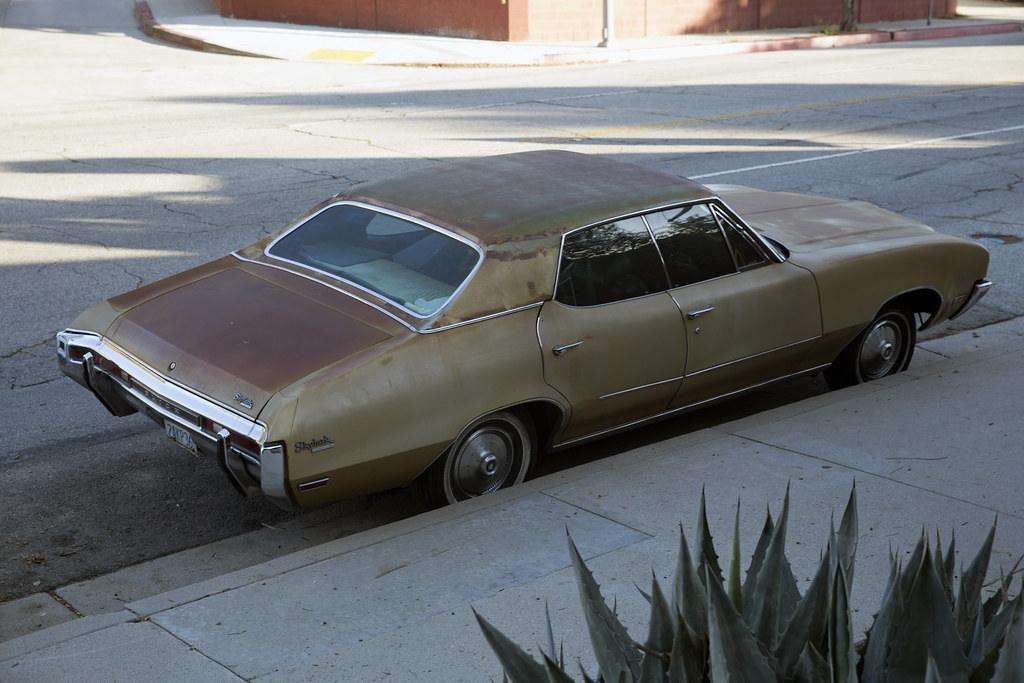The image showcases an old, beat-up vehicle, likely a Buick Skylark, parked along the curb next to a sidewalk. The once green car now appears rusty, with substantial brown and yellow rust patches, particularly on the trunk, roof, and around the windows. The car has mixed hubcaps, with a white rim on the back tire and a black rim on the front. Its side windows seem dark, possibly due to lighting, while the rear window remains clear. A small cactus plant is visible in the bottom right corner of the frame. The background features a street marked with solid white and possibly dotted lines, a sidewalk on the opposite side, and a red brick building. The scene is bathed in daylight, suggesting the photo was taken during the day, perhaps from someone standing on nearby stairs. No people or text can be seen in the image.